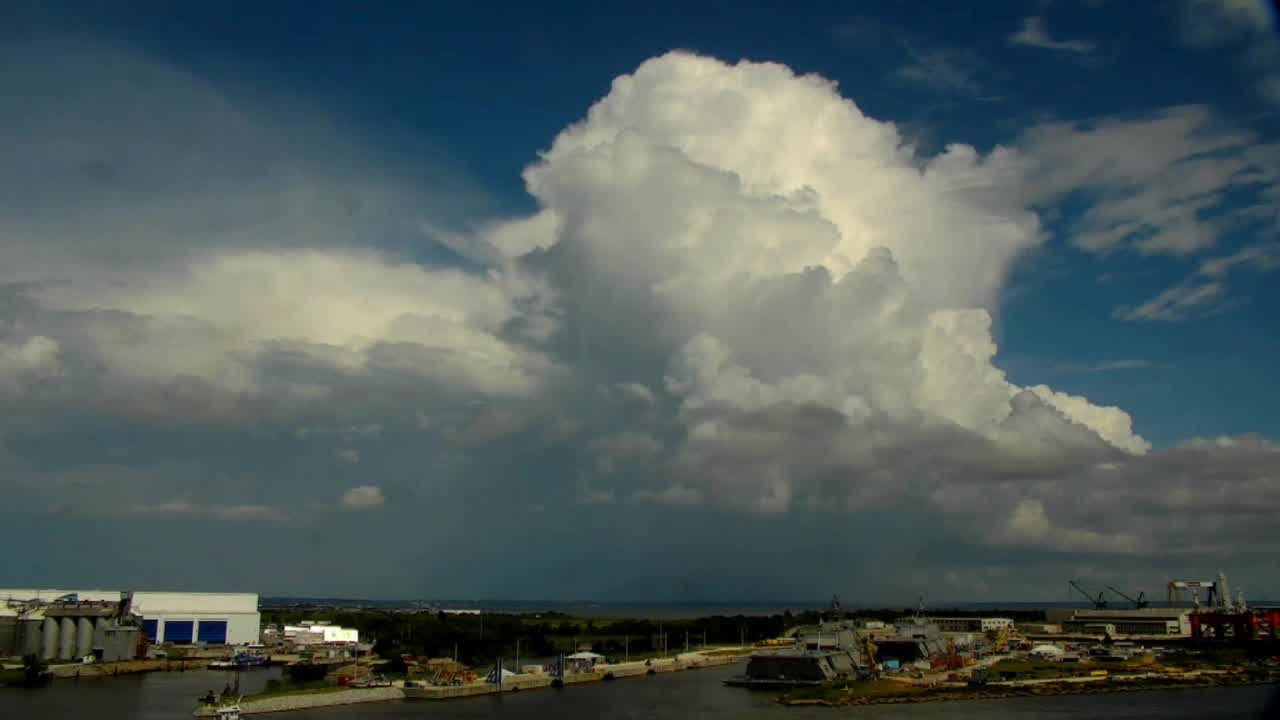The photograph depicts a dim, late-day scene at a harbor with a low horizon line, hinting that the shot was taken from a higher vantage point. Dominating the scene is a vast, dark blue sky filled with substantial, billowing white clouds. These clouds loom over an industrial landscape that presents a mix of buildings and machinery. On the left side of the harbor, a prominent white building stands alongside what appear to be factory smokestacks, with a smaller white building visible in the distance. Below these structures and scattered throughout the water are grassy islands. The right side of the image features another industrial area with distinct buildings, including a factory equipped with two cranes. The entire scene feels subdued, with the lower section of the image cloaked in shadows, accentuating the overcast atmosphere. Behind the buildings, at the water's edge, a row of trees appears bathed in shadow, adding to the scene's dim, industrial ambiance.